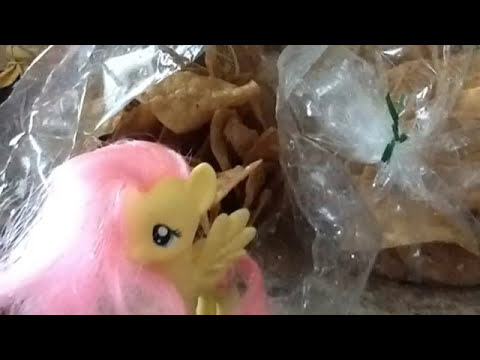The image is a full-colored horizontal photograph with a black border at the top and bottom. Dominating the lower left of the image is a small child's toy, specifically a yellow My Little Pony. This toy features notable details such as wings, blue or black eyes, and long, thick pink hair cascading off to one side, covering one eye. Also visible is a long pink tail. Nearby, almost at the center of the image, is a clear cellophane bag that appears to have been twisted shut and secured with a green twist tie, though the bag has been ripped open, revealing its contents, which seem to be either plain tortilla chips or possibly ginseng roots. Adding to the complexity of the scene is an unidentifiable brown leafy object near the center.